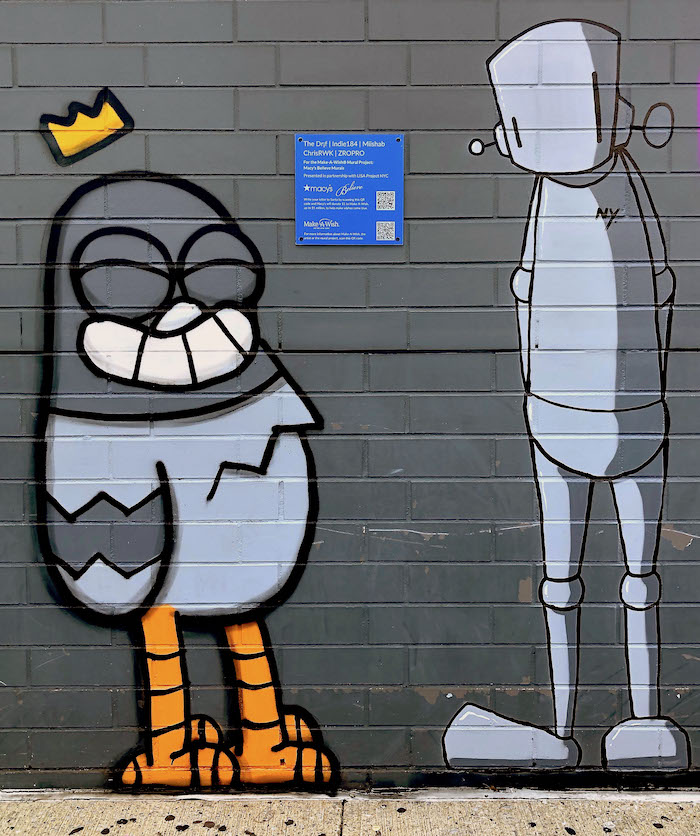The image features a dark gray painted brick wall adorned with intricate graffiti art. At the center of the wall, there is a whimsical depiction of an animal-like creature that resembles a bird, possessing gray feathers akin to a pigeon or penguin. The bird-like figure has striped legs similar to those of a chicken or duck, yellow feet with large toes, and is embellished with a floating yellow crown above its head, adding an element of surrealism. Additionally, the bird has its eyes closed and displays a broad, toothy grin.

To the right of this avian creature stands a robot-like figure, rendered entirely in shades of gray and accented with black outlines. The robot, characterized by its large feet and minimalistic face, features two prominent rectangular slots where eyes would be. Both figures complement each other with their detailed black outlines.

In the background, scattered pieces of signage and text adorn the wall, some of which include names and phrases like "Indy 184," "Mishab," "Chris RWK," "ZRO," "PRO," "Macy’s," and "Make-A-Wish," accompanied by black and white scan codes. There is also a small, blue sign with white text that is indecipherable due to its distance and the minuscule font size. The entire scene is a blend of artistic expression and urban storytelling, creating a visually compelling tableau.